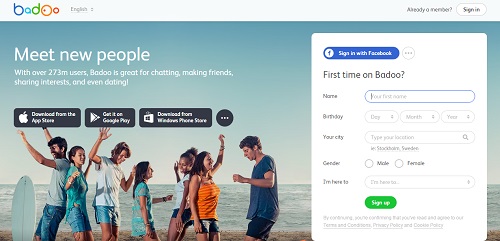In this image, we observe a screenshot from the Badoo website, as indicated by the colorful logo situated in the upper left corner. The logo features a gradient of blue, green, yellow, red, and orange hues. Adjacent to the logo on the right, there's a language selection bar currently set to English. On the far right side of the header, there is a "Already a member?" prompt accompanied by a sign-in button.

The main portion of the image showcases a vibrant beach scene with people enjoying the shoreline, with the water and sandy beach visible in the background. Superimposed on this backdrop is a prominent text that reads, "Meet new people. With over 2237 million users, Badoo is great for chatting, making friends, sharing interests, and even dating."

Below this text, we see icons indicating that the Badoo app is available for download on the Apple Store, Google Play Store, and Microsoft Store. To the right of these icons, there's a sign-up box inviting new users to fill out their information and join the platform.

Overall, the image effectively communicates Badoo's global reach and diverse functionality, encouraging users to engage with the platform for various social interactions.